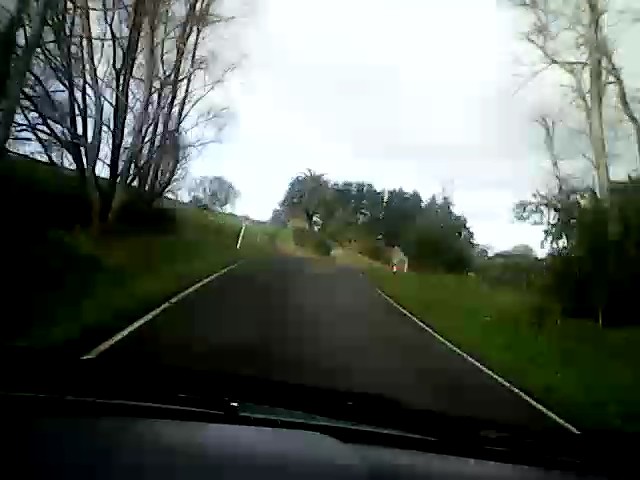The image depicts a blurry, low-resolution photograph, likely taken from the dashboard or windshield of a moving car. The central focus is on a single-lane, black asphalt road bordered by white lines. Alongside the road is greenery with green grass and tall, mostly leafless trees, suggesting an autumn or wintry setting. The road leads towards the horizon where a house or group of houses is partially visible among a cluster of trees. The sky appears bright white, possibly due to heavy cloud cover. The overall composition is blurred, with noticeable pixelation affecting the clarity of the image.